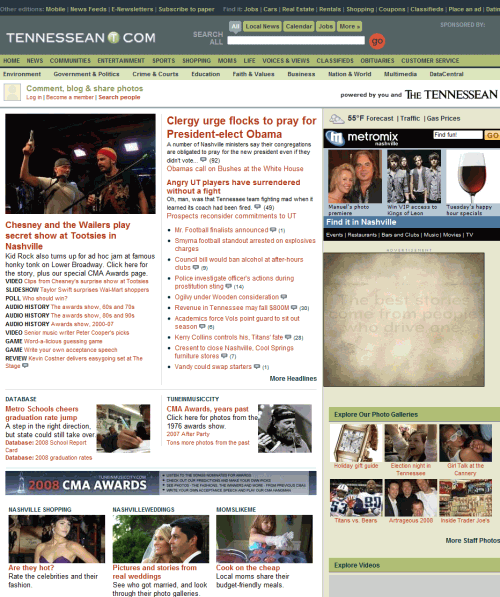This image is a detailed screenshot from a news website, Tennessean.com. At the very top, the header features a dark gray background with the publication name prominently displayed in white capital letters. The "dot" in Tennessean.com is stylized as a large green circle. To the right of this logo, there's a long, white rectangular search box. Above the search box, a navigation bar includes categories such as "Latest News," "Calendar," "Jobs," and "More," with "More" indicated as a drop-down menu. 

Above this header, there is a narrower black border with additional menu items that are unfortunately too small to read. Just below the main header, a secondary menu with a green background offers further navigation options including "Home," "Jobs," "Companies," "Entertainment," "Sports," "Shopping," "Voices and Views," "Classified," "Obituary," and "Customer Service."

The main content of the webpage displays the news items. The central column features a headline in red, proclaiming "Clergy urge flocks to pray for President-elect Obama," dating the screenshot to 2008. On the left side of the page, a photograph is accompanied by the caption: "Chesney and the Wallers play in secret show at Tootsies in Nashville."